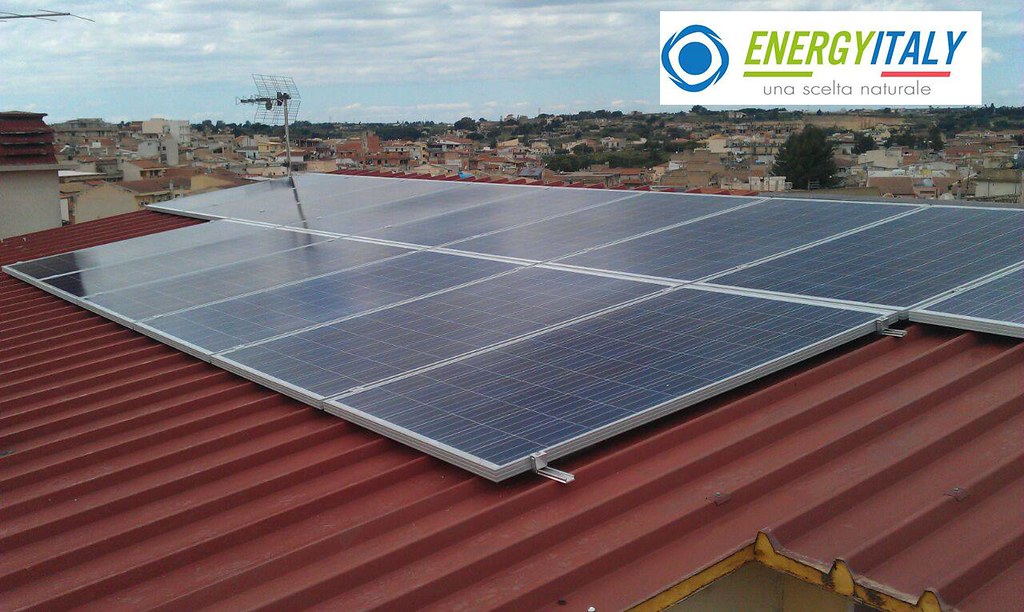This photograph, likely part of an advertisement for a solar power company, captures a detailed scene taken from a rooftop. The roof, composed of red metal sheets, features an installation of approximately 12 to 14 black solar panels framed in gray metal, lined up in sections. In the top left corner of the roof, a television antenna is visible. The backdrop reveals a descending hillside dense with houses, many of which have red tile roofs, indicating the setting is within a town. The sky above is mostly cloudy with white, gray, and black clouds, though some blue is peeking through, giving an overcast feel to the day. In the top right corner of the image, a white rectangular sign displays the logo and text of "Energy Italy" in blue and green, with the phrase "Una Scelta Natural" in light gray, all elements pointing to the branding and likely promotional nature of the photograph.